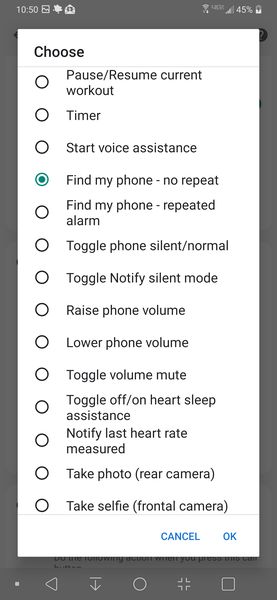A detailed screenshot from a smartphone interface showcases a wealth of information and options. At the top, the status bar reveals the current time, open app indicators, various notifications, Wi-Fi signal strength, data signal, and battery percentage. Central to the image is a prominent white pop-up box bearing the title "Choose" at the top, followed by an extensive list of radio button options. These options include: 
- Pause/Resume Current Workout
- Timer
- Start Voice Assistant
- Find My Phone - No Repeat (selected)
- Find My Phone - Repeated Alarm
- Toggle Phone Silence/Normal
- Toggle Notify Silent Mode
- Raise Phone Volume
- Lower Phone Volume
- Toggle Volume Mute
- Toggle Off/On Heart Sleep Assistance
- Notify Last Heart Rate Measured
- Take Photo (Rear Camera)
- Take Selfie (Front Camera)

At the very bottom of the pop-up box are two buttons labeled "Cancel" and "Okay." Below the pop-up box, the smartphone's navigation bar is displayed, featuring icons for back, download, home, minimize, and an unidentified function. The background of the phone behind the popup is a dark gray color, providing contrast to the bright white of the dialog box.